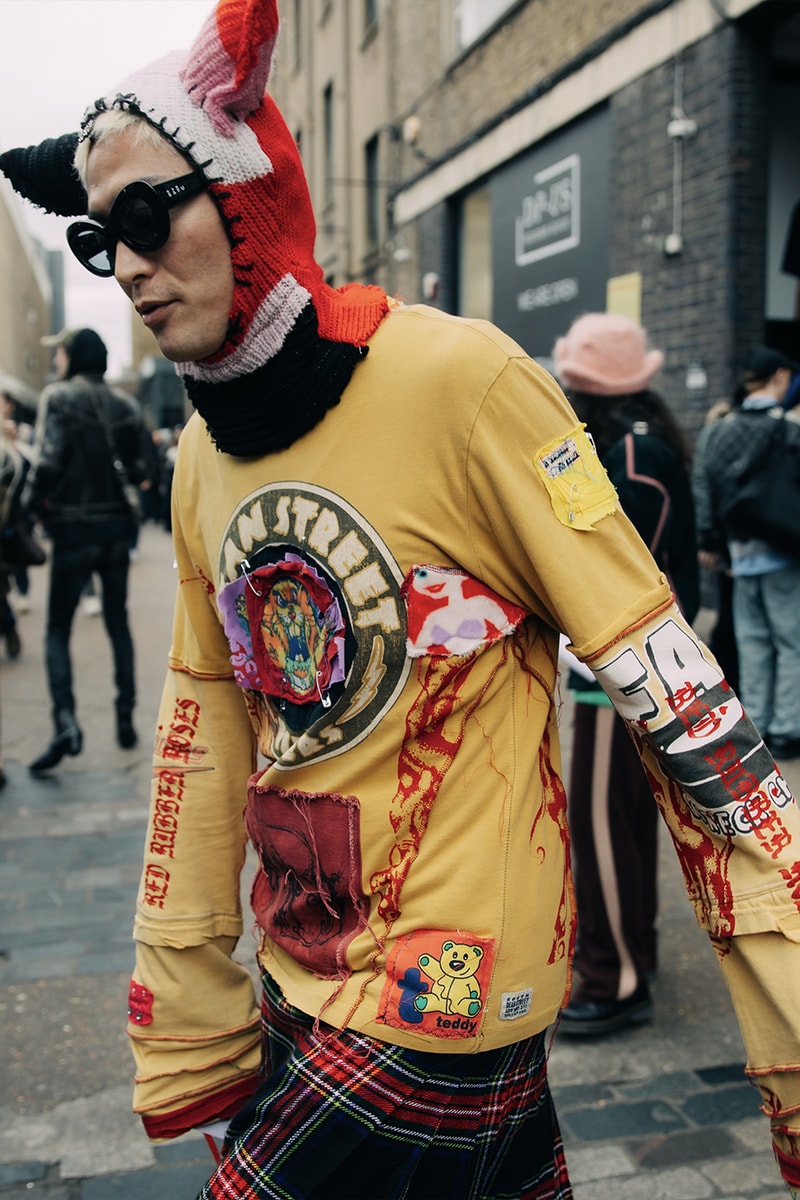In this live photograph taken in portrait mode, the background features a somewhat blurry, tan-colored cityscape with dark black bricks at the top and various shades of tan and brown cement below. People and buildings can be faintly seen in the background, along with the sky. In the foreground, a male figure is the primary focus, walking towards the left. He dons a vibrant and whimsical hoodie with pointed ears resembling an animal, featuring a color palette of red, white, pink, black, and orange. His left ear is notably black. The hood drapes down to a scarf-like attachment around his neck. His face, partly obscured by a pair of black sunglasses—one lens completely opaque and the other see-through—reveals short blond hair peeking out. 

His attire includes a striking long-sleeve yellow shirt adorned with a multitude of eclectic patches: a circle on the front possibly reading "A.N. Street" with the word "STREET" encircled in yellow, a snippet of an orange-haired mermaid, a red patch, and various other quirky and colorful designs, including a cat with sharp teeth and the Tasmanian Devil. Both sleeves of his shirt are inscribed with the words "red rubber roses." Complementing this, he wears a primarily green plaid skirt with red and yellow stripes, mistaken in some accounts for Scottish tan bottoms or a kilt.